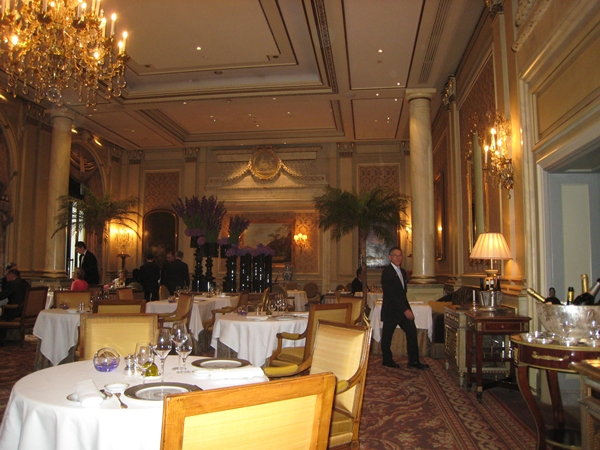The image depicts an opulent banquet hall or high-end hotel restaurant, adorned with elegance and sophistication. Round tables dressed in crisp white tablecloths are set with wine glasses, plates, and cutlery, while cushioned chairs in a yellowish-beige, gold-like hue surround them, lending a luxurious feel. A man in a black suit is prominently seen walking towards a door, with a bucket of champagne seated on a nearby table. The background reveals well-dressed individuals, some in black suits and a woman in pink, either seated at tables or standing to the left side of the room. Grand gold chandeliers with lit candles illuminate the space, and it's further accentuated by white ceilings and cream-colored marble columns flanking both sides of the room. Large, strategically placed plants, includings palm trees and purplish flowers, add to the opulence. A rich, burgundy or red rug graces the floor, tying together the extravagant decor of this well-established, expensive restaurant.